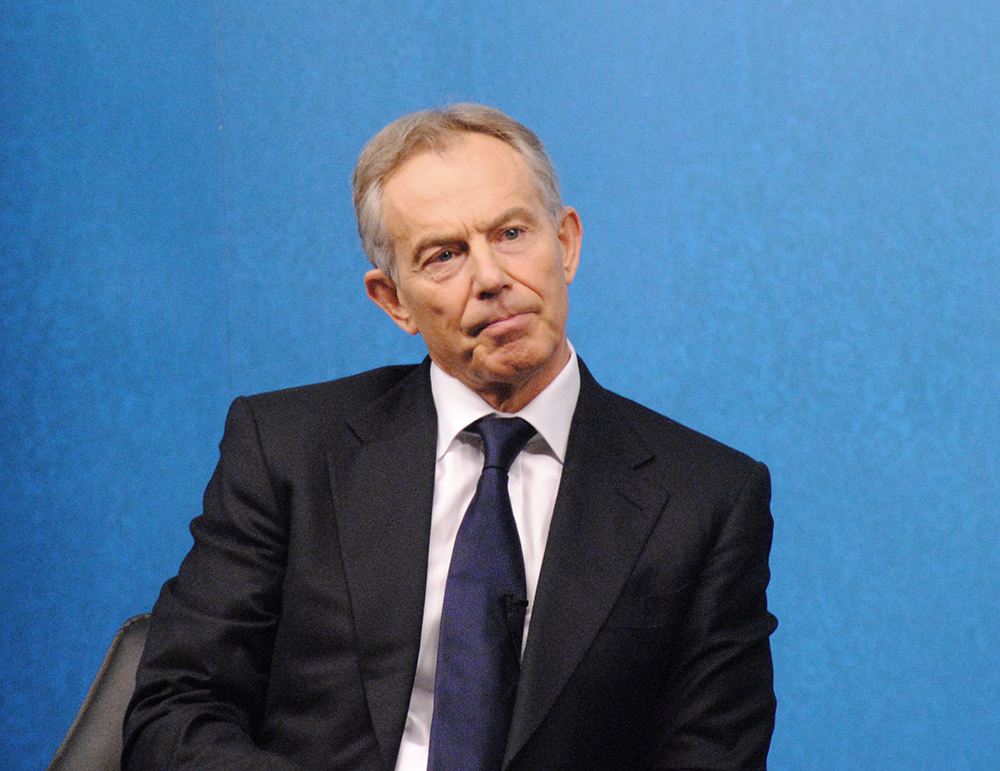The image depicts a well-groomed older gentleman, possibly a politician resembling former UK Prime Minister Tony Blair, seated and facing forward. The photograph captures him from the stomach upwards, revealing a black suit jacket over a white shirt and a dark navy blue tie. His short gray hair is neatly styled, and he appears contemplative, gazing slightly to the right with his head tilted. A small black microphone is clipped to his tie, suggesting he might be in an interview setting. The edge of a black leather chair is visible on the left side of the image. The background is a solid light blue, and the image is sharply lit and clear, presenting the subject in a professional and composed manner.